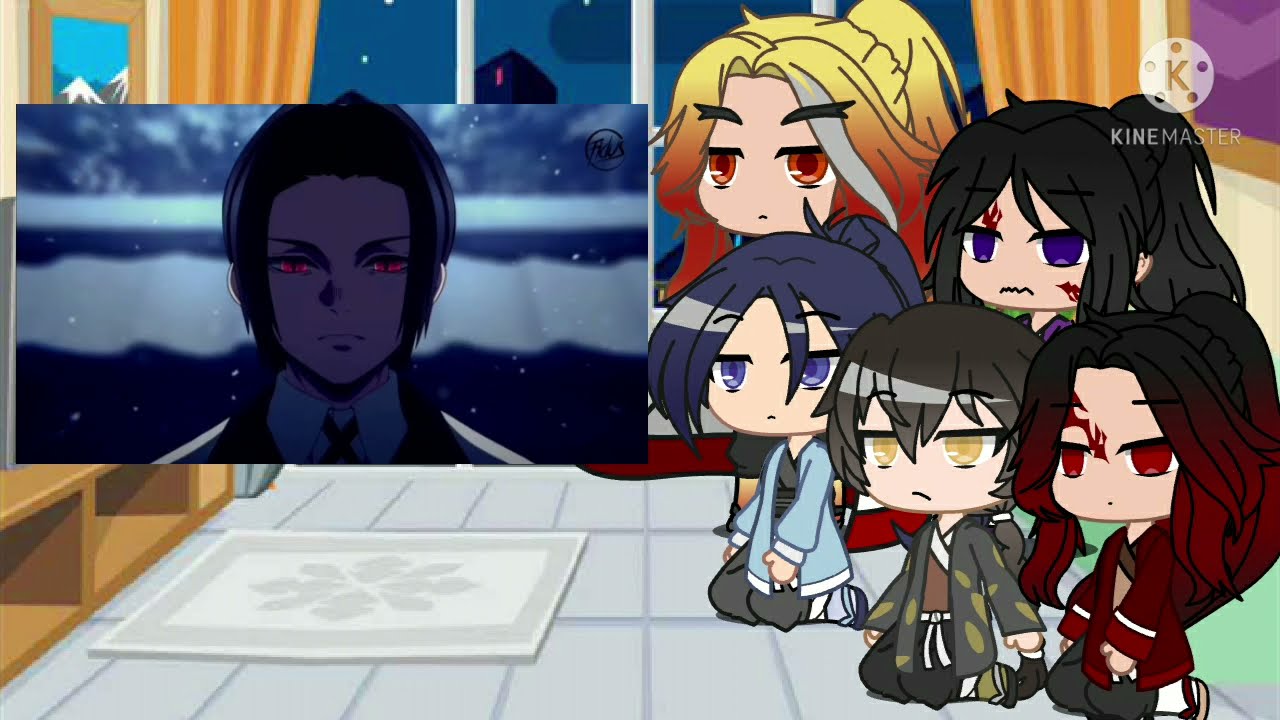The image is a vibrant and detailed scene featuring five anime-style characters on the right side, kneeling on a tatami mat. These characters, who possess a variety of hair colors and styles that match their outfits, are intently gazing at a separate inset image on the left. In this inset, a serious-looking man with red eyes and dark short hair, possibly from another anime or video game, appears on what looks like a TV screen, given the contrasting art style and color tone. The inset image has a blue background with snow, making the man's red eyes stand out even more, and he is wearing a collared white shirt with a tie. Among the group of five characters, there is a girl with blonde hair transitioning to red at the tips, wearing red and possessing red eyes, a girl with black hair and purple eyes, another with black hair with red tips and red eyes, one with gray hair and yellow eyes, and finally, a girl with blue hair and blue eyes wearing a blue shirt. They all have large, expressive eyes typical of anime style. The background includes a pale blue floor with an area rug, adding to the cozy, indoor setting. Additionally, there is a "Kinemaster" logo with what looks like an old film reel in the upper right-hand corner of the image.